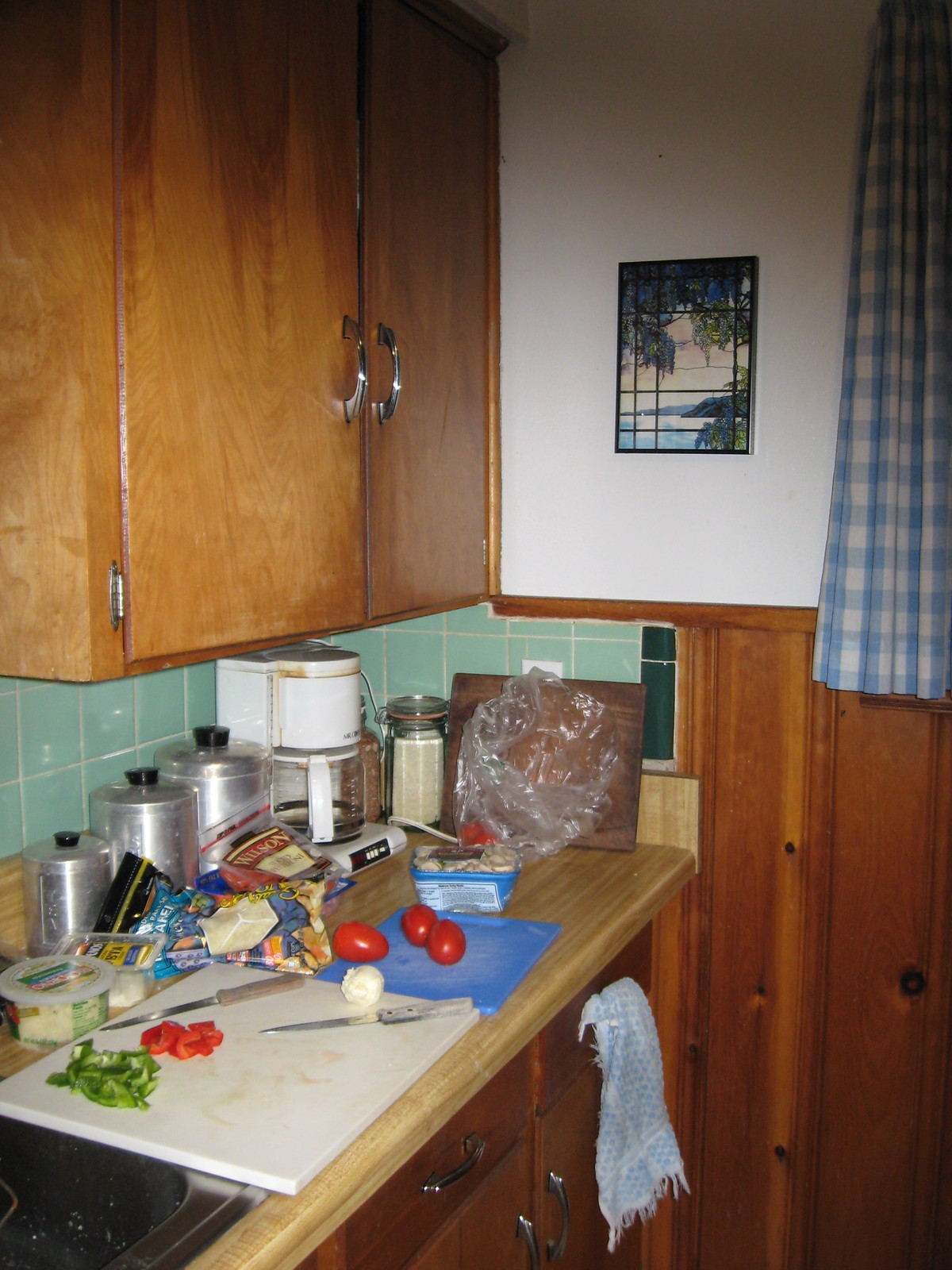A detailed image of a well-organized kitchen features wooden cabinets with sleek silver handles, present both above and below. The light wooden countertops hold a white cutting board adorned with chopped lettuce and tomatoes, along with a couple of knives. A trio of untouched tomatoes rests on a separate cutting board nearby. Against one of the walls, another cutting board leans casually. The backsplash showcases a tile picture depicting an outdoor scene. To the side, blue and white plaid curtains frame a window, while a black sink is partially visible on the left. Various tins with closed lids are neatly arranged against the wall, and a package of mushrooms sits on the counter, hinting they might soon be chopped, possibly for a salad. The countertop holds an array of kitchen essentials, suggesting active meal preparation in progress.